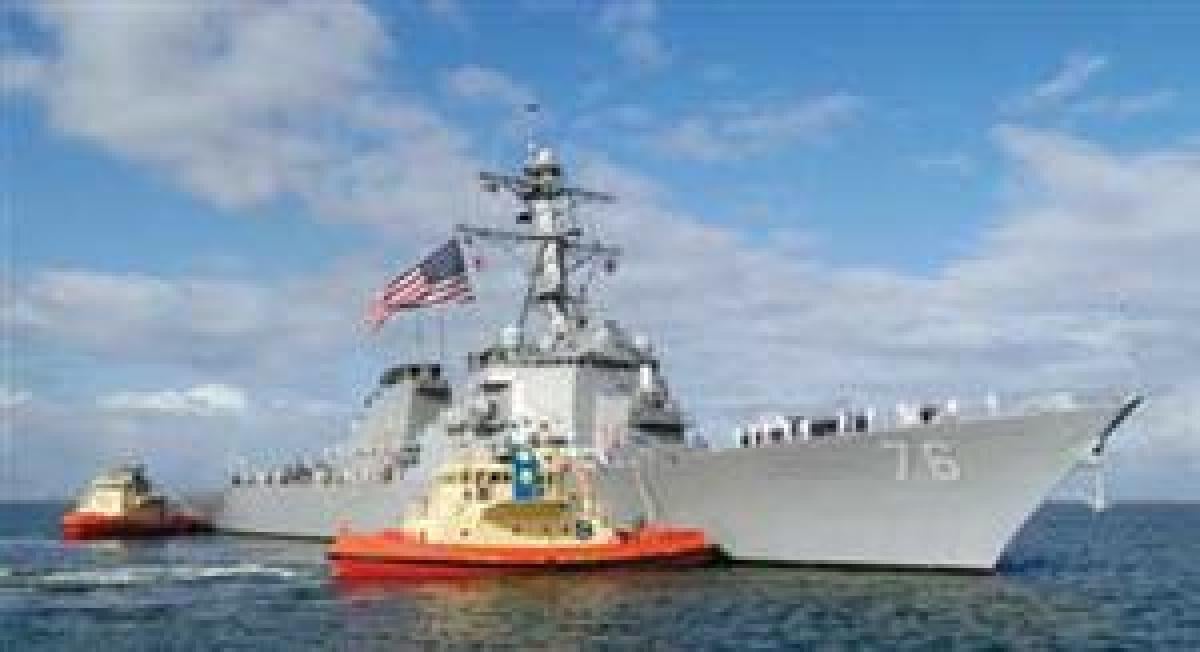In this grainy and pixelated daytime photograph, a large gray U.S. Navy warship, marked with the number 76, is seen floating in the ocean. The ship prominently displays an American flag that waves in the wind. Accompanying the ship are two small high-visibility boats, featuring orange bottoms and yellow-tops. These boats appear to be either aiding the larger vessel or attempting a boarding procedure. The backdrop consists of a grayish-blue ocean with several clouds scattered across a light blue sky. The overall image quality is quite low, which makes the photograph appear blurry and lacking in fine detail.